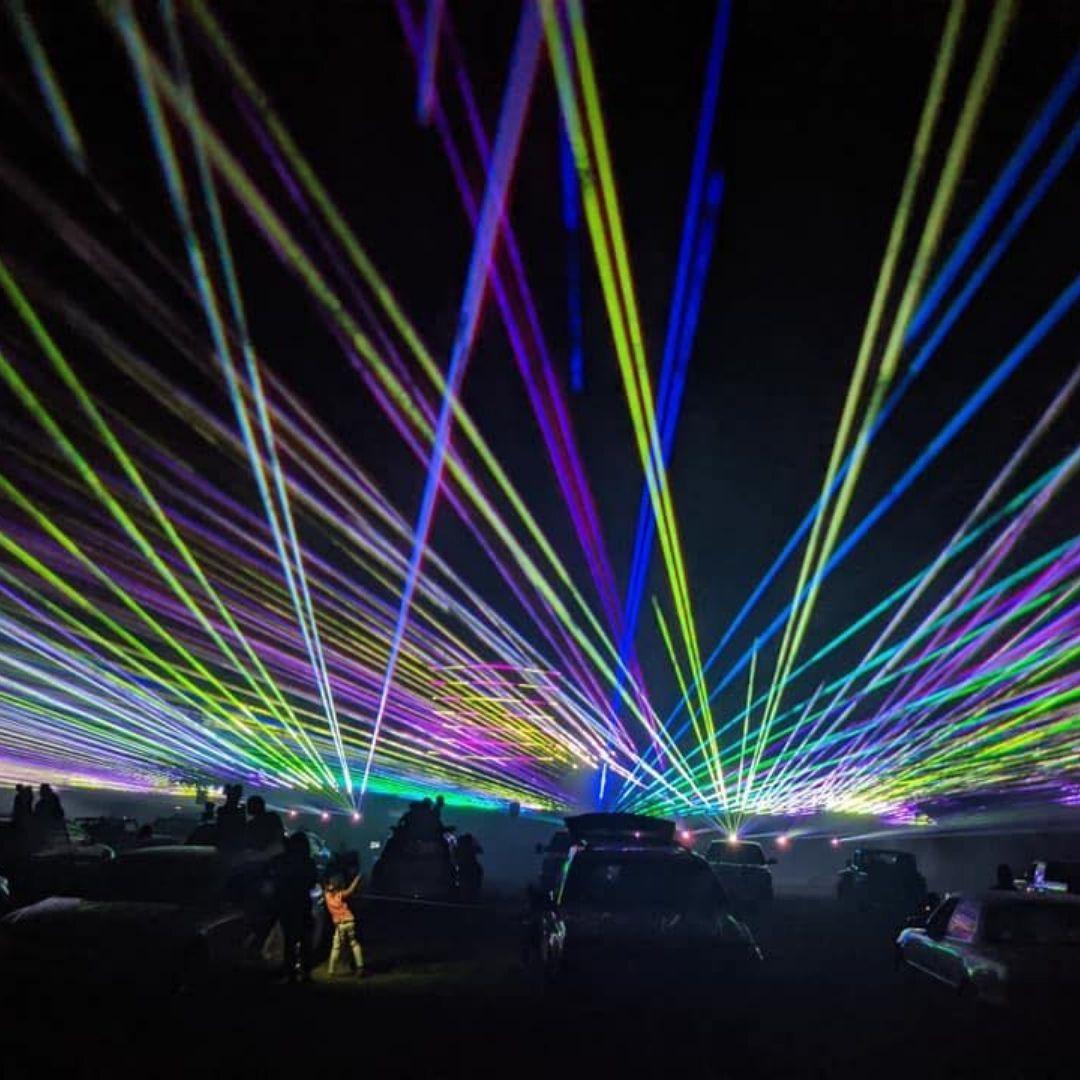In this captivating nighttime scene, dozens of cars are parked semi-circularly or in clusters under an almost pitch-black sky, their dark silhouettes barely visible. Among these cars, silhouettes of people are standing around or sitting on top of their vehicles, all focused on the breathtaking laser light show overhead. Streaks of vibrant blue, purple, yellow, and green laser beams form a dazzling dome-like spectacle in the sky, emanating from several glowing projectors in the background. Over a hundred laser beams shoot across the night, creating a mesmerizing display. Adding to the lively atmosphere, a person in an orange shirt can be seen dancing amidst the cars, their figure illuminated by the brilliant laser lights.